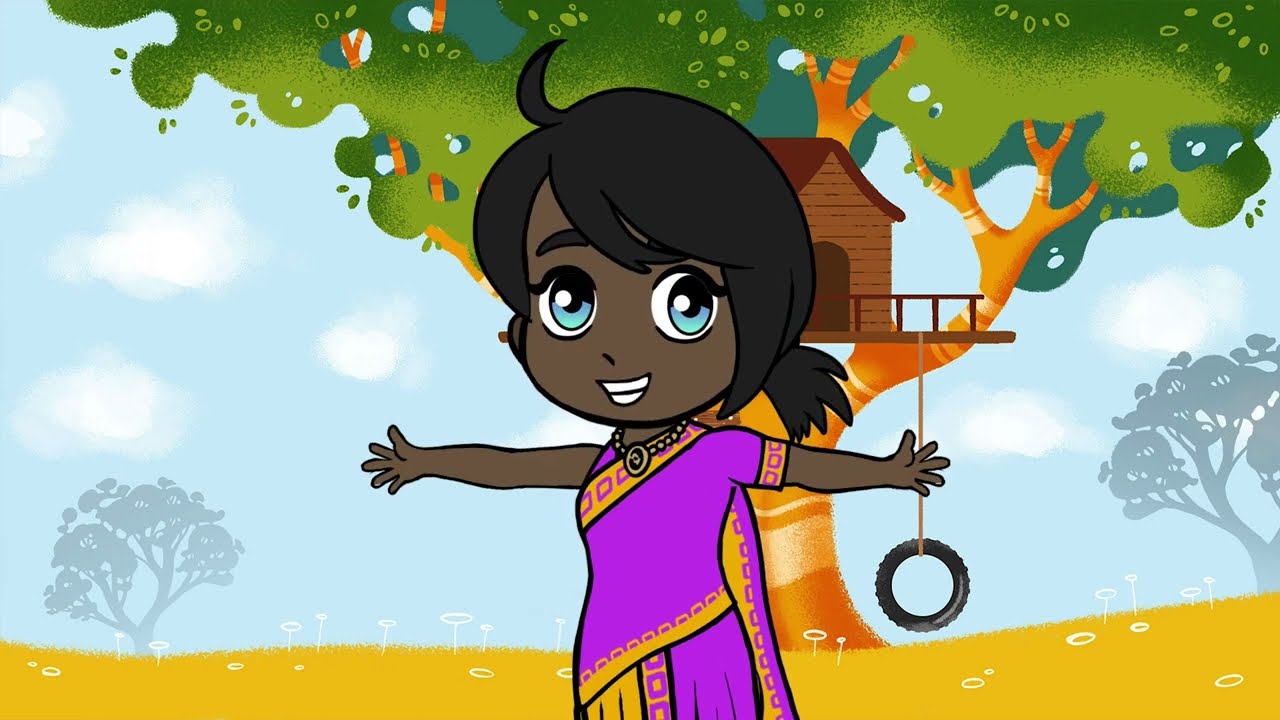The image depicts a cartoon of a young, dark-skinned Indian girl with bright blue, circular eyes, black hair styled with bangs and a short ponytail, and a small, white-toothed smile. She is dressed in a purple sari adorned with yellow borders and gold accents. The setting behind her features a golden expanse of grass dotted with white flowers, under a clear blue sky with many fluffy white clouds. Prominently in the background stands a large tree with golden bark, hosting a treehouse and a black tire swing hanging below it. Additional trees are outlined behind the main tree, completing the picturesque scene.